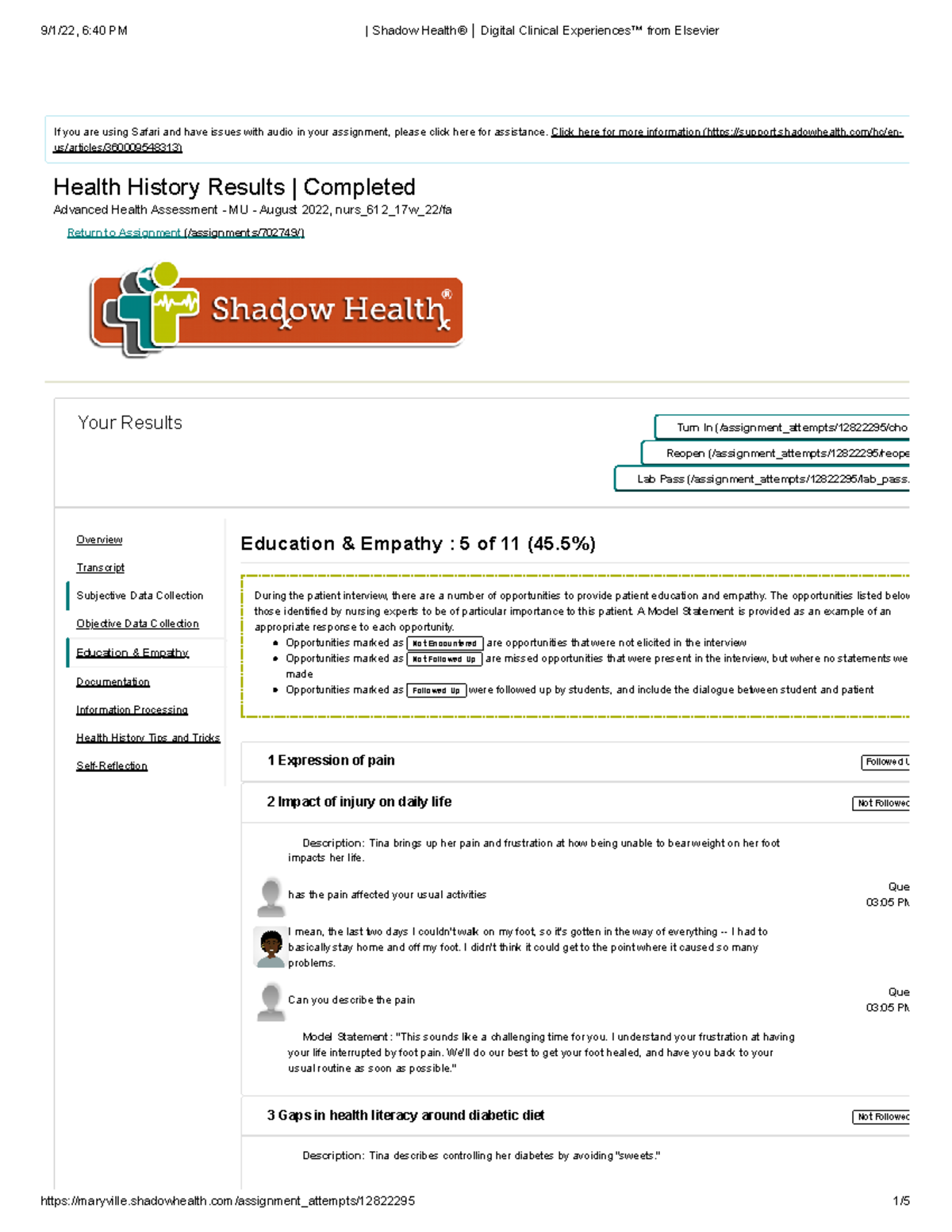This image is a screenshot of a website or application, presented in a portrait orientation, approximately twice as tall as it is wide. The background is predominantly white with black text, featuring minimal color accents. At the top, there is a rectangular, horizontal button in orange with white text that reads "Shadow Health." Adjacent to this button is a logo comprised of three stylized outlines of people, sequentially colored in purple, blue, and light green. The frontmost light green figure includes a white line that resembles a heartbeat monitor.

Above this logo, there is text stating "Health History Results Completed," and directly below it is a section titled "Your Results." The visible portion of this section includes a header for "Education and Empathy," specifying the completion status as "5 of 11, 45.5%." Further content is visible beneath this header, though the text is too small to read clearly. This lower section is predominantly text-based and includes three avatar head-and-shoulders icons to its left; two are blank gray, indicating placeholders, while one is more detailed, suggesting an active or selected state.